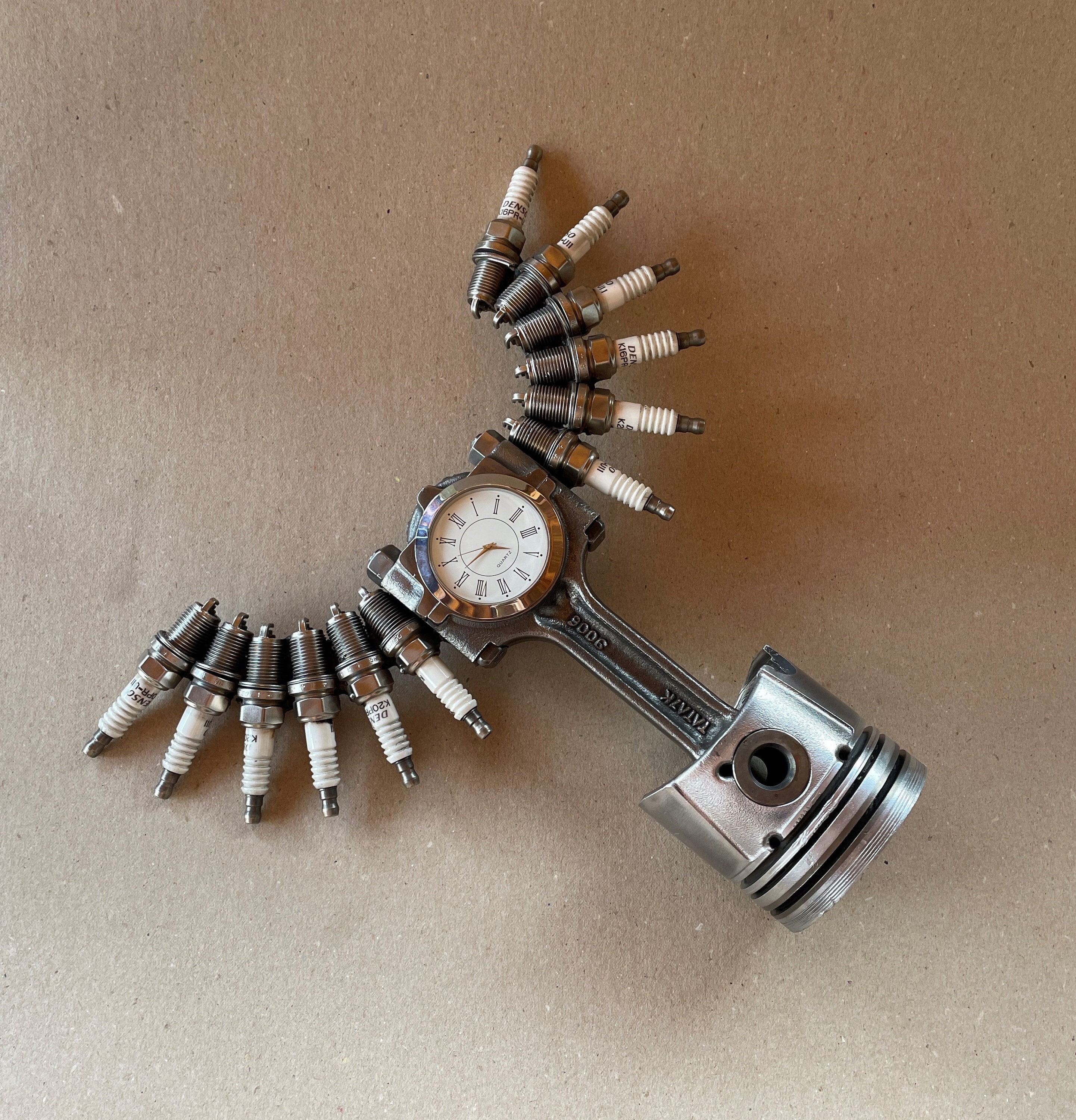The image features an intricately designed piece of metalwork art laid against a gradient background that transitions from a grayish pink at the bottom to a very dark pinkish-white at the top. The object itself has a silver tube with a rounded cup-like bottom which might resemble a cap with a black hole in it, suggesting an intentional design. Extending from the tube, there is a stem adorned with six spark plugs on each side. These spark plugs have white bases and silver tops, fanning outwards and upwards like wings. 

At the center of the stem, there is a clock with a white face and bronzy-gold hands, enclosed with a brown outer circle. This clock is positioned where one might expect a handle if it were a spoon, contributing to the object’s unique and fascinating structure. The entire piece is small in size and crafted with various screws and bolts that accentuate its wing-like appearance. It appears zoomed in and is viewed from a diagonal angle, making it a remarkable and detailed piece of art.